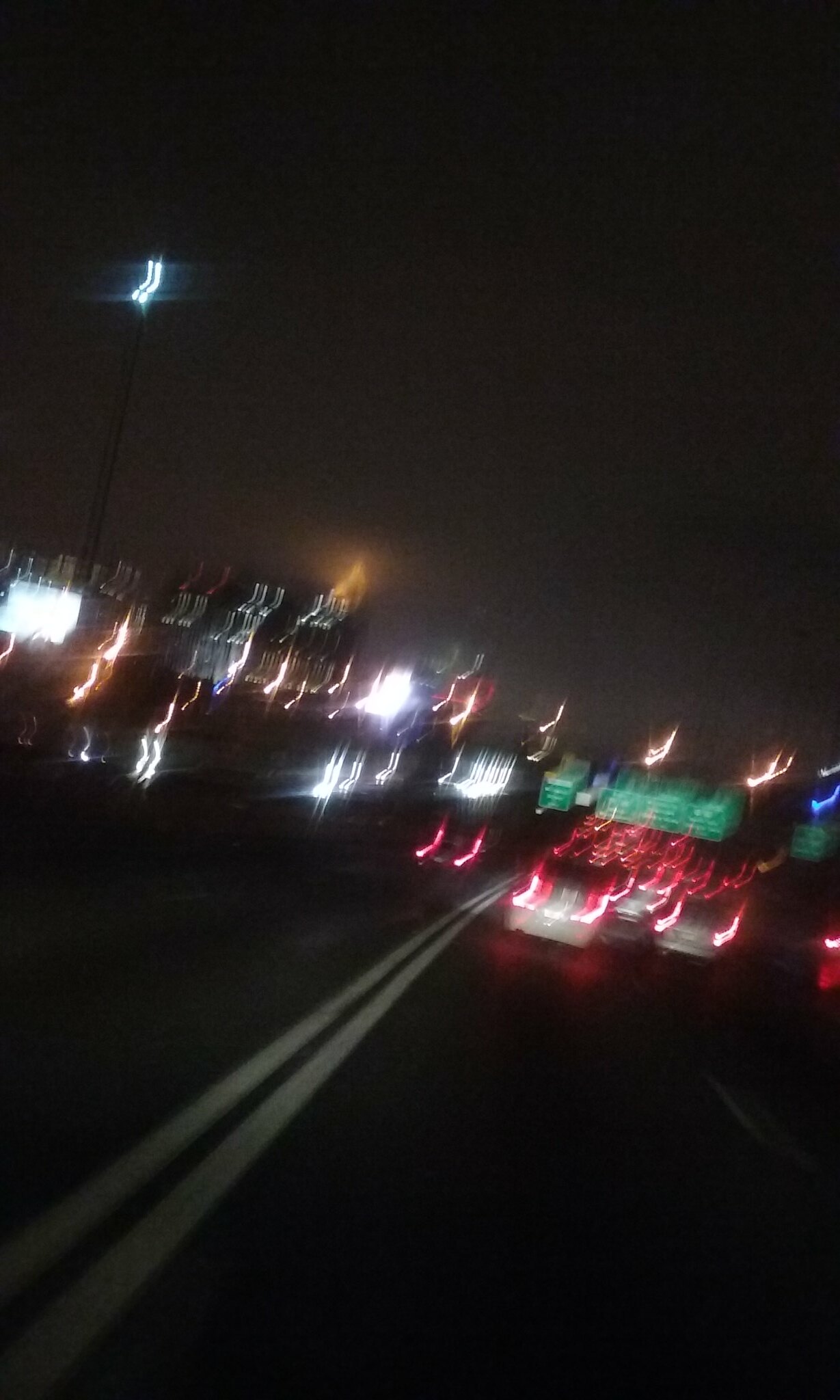The photograph captures a nighttime scene on a busy freeway, enveloped in darkness with blurred lights adding to the dramatic atmosphere. Central to the image is a two-lane marker running down the middle of the road, clearly delineated despite the dim lighting. Directly in front of this marker, a dense stream of brake lights gleams from the rear of numerous cars, illuminating the path upwards through the image.

Hovering above the vehicles, two distinct road signs catch the eye. To the left, a green rectangular sign with red text provides crucial navigation information. Adjacent to it, a longer, more elongated sign is visible, marked by white text. Both signs are highlighted by surrounding street lights that punctuate the scene with halos of artificial illumination.

On the left side of the image, the headlights of oncoming traffic pierce through the darkness, adding a contrasting layer of light. Behind this oncoming traffic, city elements like street lights and the illuminated windows of buildings dot the background, adding depth and context to the urban setting. The overall composition vividly captures the bustling yet somewhat chaotic essence of a nighttime freeway.